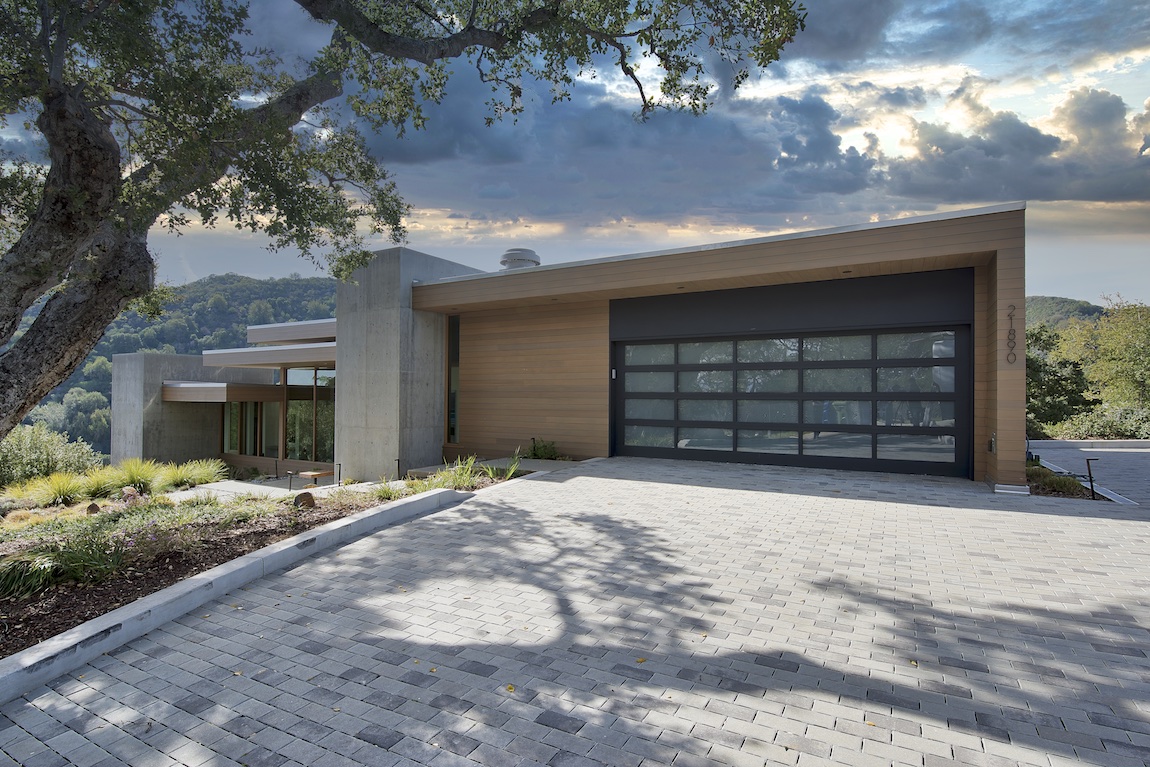This image captures a striking modern contemporary home built atop a hillside, viewed from the expansive gray stone paver driveway. The home features a square architecture, combining wooden sections and concrete substrates on its exterior. Dominating the front facade, the garage door is fashioned from glass with black metal frames and is flanked by a massive cinder block column to its left. Above the garage, a brown awning complements the brown wood paneling and the extensive glass walls reflect the surrounding trees. In the background, a mountain range stretches horizontally, under a sky filled with layering gray and white clouds, with a touch of orange sunlight peeking through. A large, diagonally tilted tree with green branches occupies the left side of the image. The setting suggests a remote and upscale location, likely designed by a renowned architect.